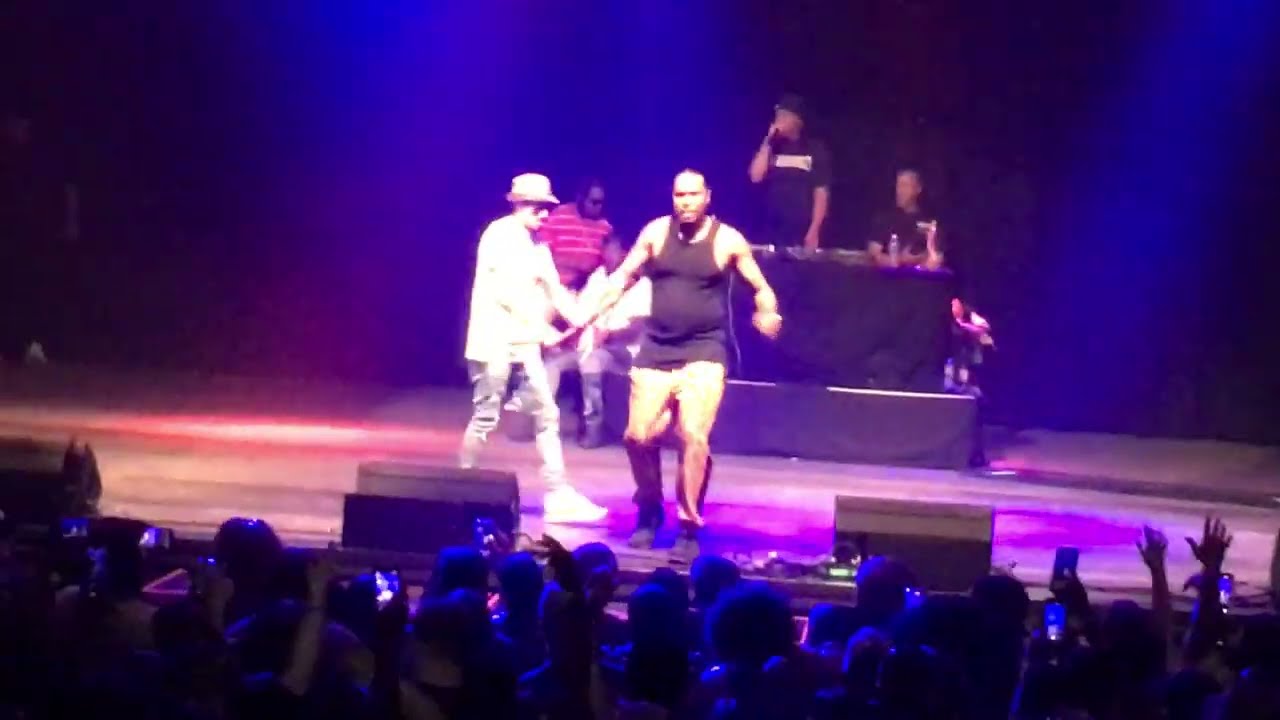The image captures an energetic concert scene, viewed from within the crowd. The foreground is filled with rows of silhouetted audience members, their heads popping against the bluish-purple tint provided by the stage lights. Many are raising their hands and some are holding cameras, immersed in the musical experience. On stage, a central figure, an African-American man clad in a black tank top and tan pants, stands prominently. He appears to be overweight, with his knees bent and arms at his sides, engaging with the audience. To his left (or possibly right from the viewer’s perspective), another performer wearing a long-sleeved white shirt, a light-colored hat, ripped jeans, and white sneakers walks toward him, almost as if reaching out.

In the background, an elevated black table serves as a DJ booth. One man stands behind it, microphone in hand, addressing the crowd, while another sits nearby. Additional figures are faintly visible on stage, contributing to the lively atmosphere. The stage itself is bathed in a blue hue, contrasting sharply against the dark backdrop. Meanwhile, lights of various shades—reddish, purplish, and blue—stream and reflect off the stage and onto the captivated crowd, creating an electrifying ambiance. Overall, the image evokes a sense of unity and excitement, with people dancing and enjoying the performance.